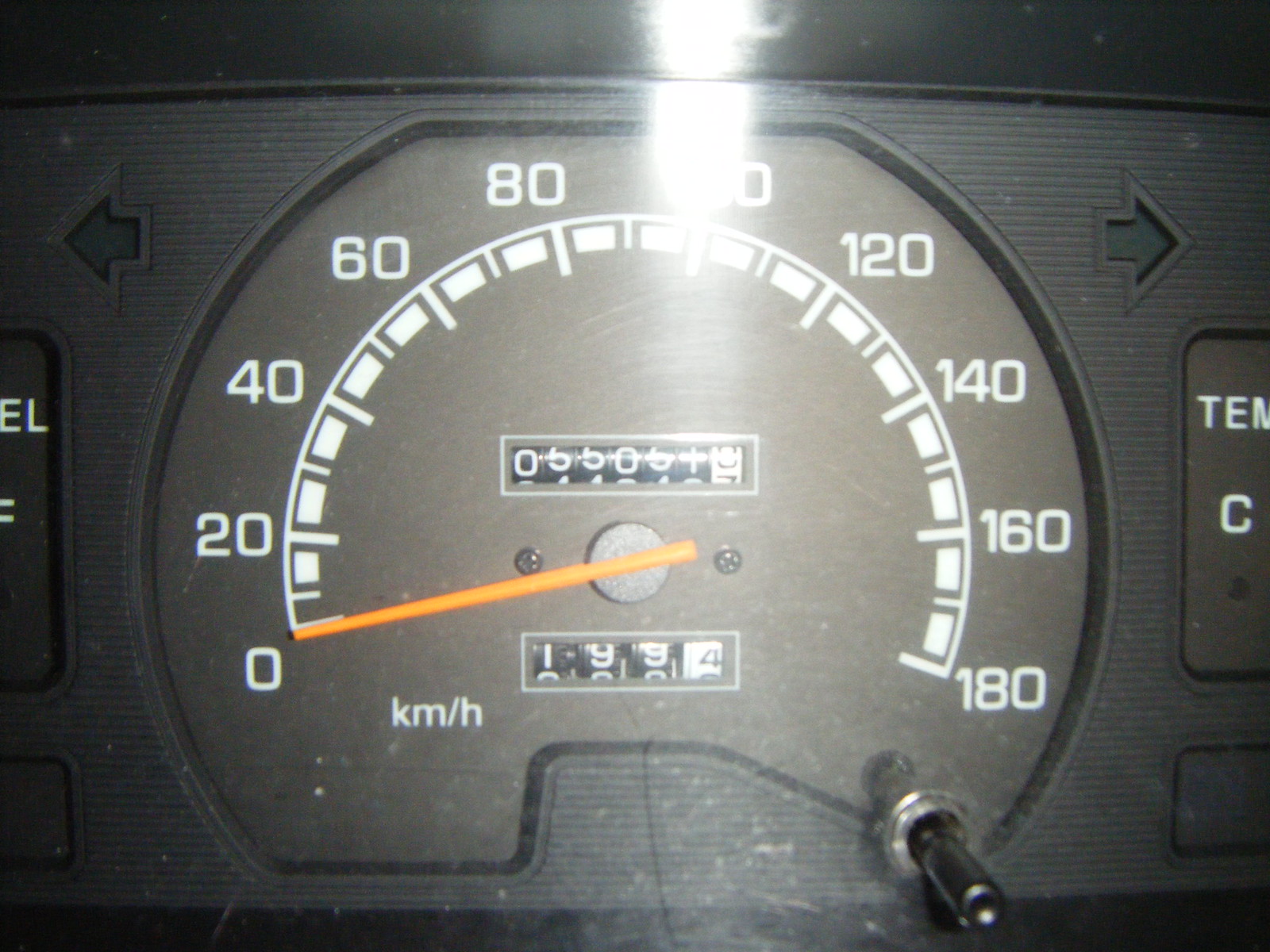The image features a close-up of a car speedometer which dominates the frame, rendered in a sleek black design. The speedometer is symmetrically flanked by left and right turn signal indicators. At the center of the speedometer, a large semicircular dial showcases white numerals ranging from 0 to 180, increasing in increments of 20. These numbers are underscored by a white semicircle with fine lines and small white rectangles marking each increment.

In the middle of the speedometer dial, a rectangular digital display shows mutable numbers, indicating the vehicle's current speed in a digitized format. At the moment captured, the digital numbers appear to be in transition, depicting "5", "4", "0", "5", with the digit "2" somewhat obscured due to a glare.

A thin, orange needle extends from the center of the dial and is presently pointing towards 0, indicating the car is stationary. Beneath this, another digital rectangle displays an odometer reading: "1", "9", "8", "8", and "4", with some digits transitioning between values. The bottom left corner of the speedometer face clearly spells out "KM/H", denoting the speed measurement unit in kilometers per hour.